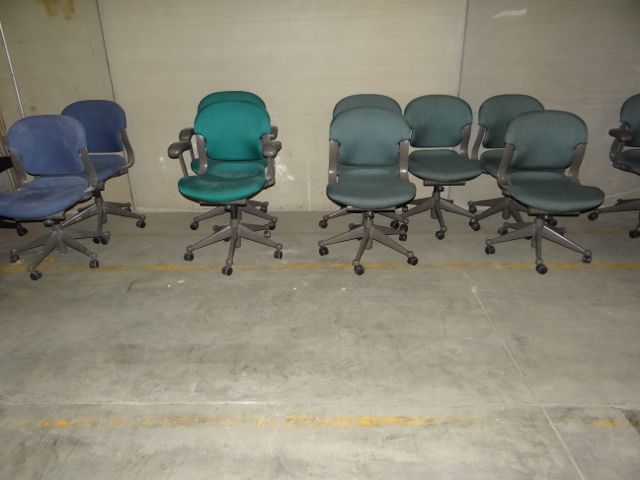In a spacious industrial warehouse with a concrete floor and walls, a collection of eleven office desk chairs is neatly arranged into three distinct color groups. To the left, there are two royal blue chairs, followed by two teal or aquamarine ones. To the right, five darker green chairs, with a hint of gray, complete the set. All the chairs feature padded seats and backs, gray armrests, and rolling claw-like bases, suggesting they are ergonomic and adjustable. A partially visible chair of a similar design sits off to the side. A yellow line on the concrete floor denotes a walkway, reinforcing the industrial setting, and a large, white sliding door interrupts the concrete wall in the background.